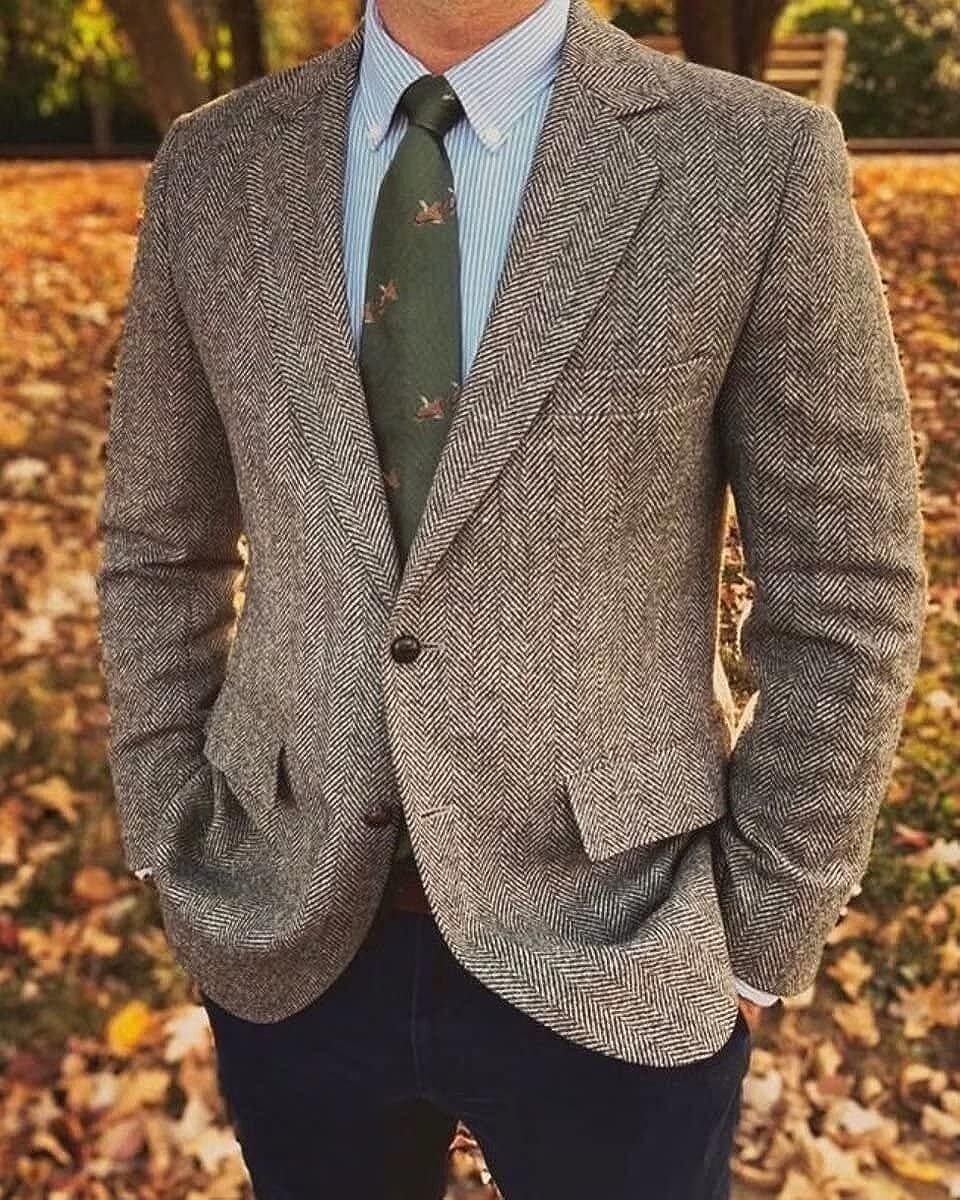A crisp, clean photograph captures a headless, centered man standing outdoors in a fall setting. His attire consists of a light brown, tweed-patterned sports jacket with a single brown button, and two pockets on the sides and one on the left side of the chest. Underneath, he wears a white shirt adorned with blue pinstripes and a dark green tie featuring small, reddish figures or prints, possibly depicting hornets or ducks. His hands are casually tucked into the pockets of his dark blue jeans, which are secured with a leather belt. The background showcases a park-like setting embellished with fallen autumn leaves and blurred tree trunks. A bench is faintly visible, adding to the seasonal ambiance of the photograph.